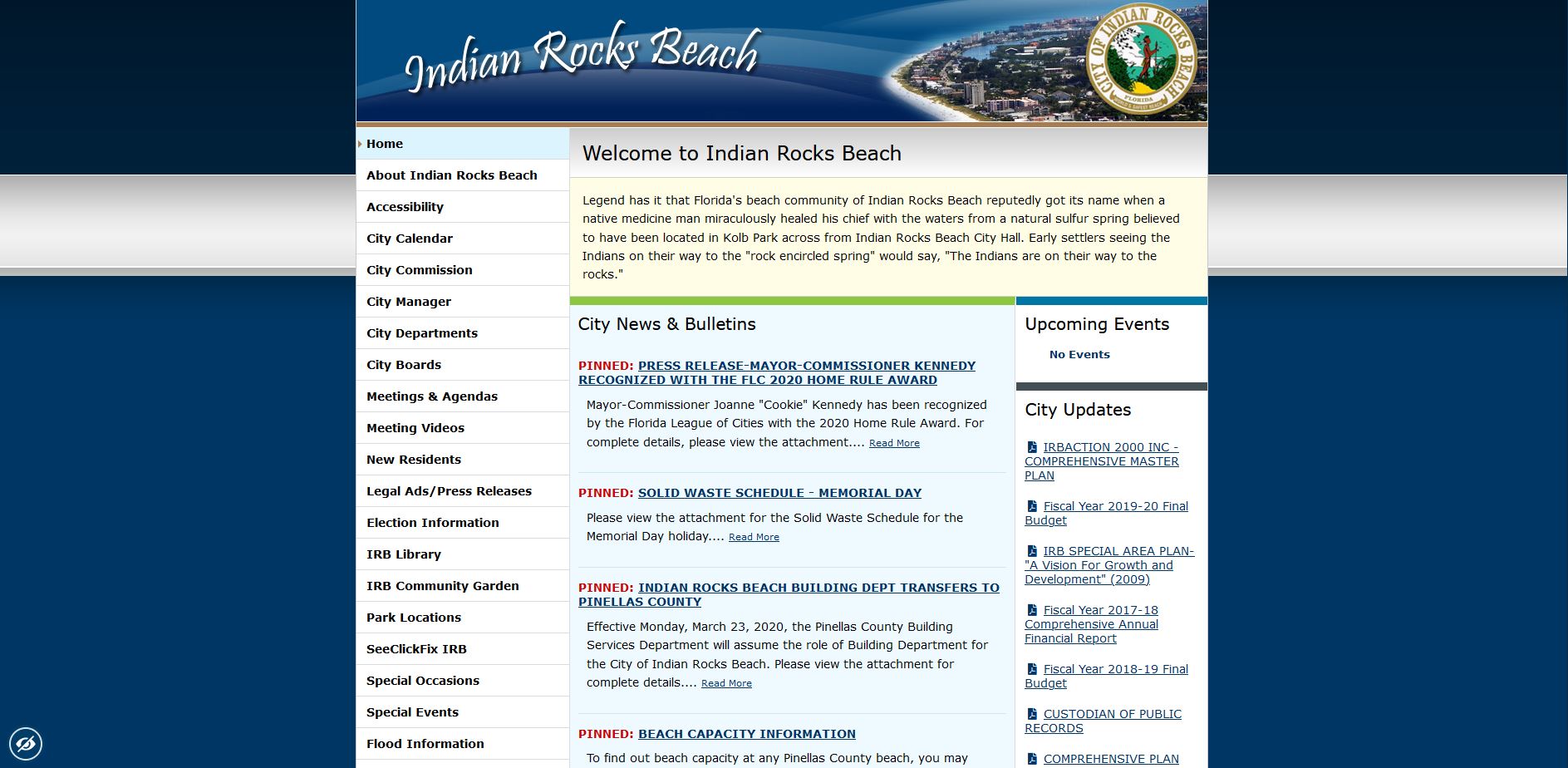Here is a detailed and cleaned-up caption for the image described:

---

The web page depicted in the image features a structured design with multiple banners and sections. The top banner is a dark blue, followed by a light grey banner, and then a lighter shade of blue banner. At the top center of the page is a blue background with white font that reads "Indian Rocks Beach." To the right of this text is an image of the beach with the town or city area visible in the background. An orange circle, or light brown circle, surrounds the text "Indian Rocks Beach" and contains a green logo that resembles a statue.

Below this section, there is a grey font that says "Welcome to Indian Rocks Beach." On the left side, there is a menu with a light blue background and black font that includes the following links: 
- Home
- About Indian Rocks Beach
- Accessibility
- City Calendar
- City Commission
- City Manager
- City Boards
- City Departments
- Meetings and Agendas
- Meeting Videos
- New Residents
- Legal Aid / Press Releases
- Election Information
- Library (IRB Library)
- IRB Community Center
- Park Locations
- See Click Fix IRB
- Special Occasions
- Special Events
- Flood Information

On the right side, there is a section for "Upcoming Events," which currently states "No events." Below this, there is a "City Updates" section, featuring several clickable links. The center of the page features "City News and Bulletins," with links for:
- Press Releases
- Solid Waste Schedule (pinned in red)
- Indian Rocks Building Department Transfers to Pinellas County
- Beach Capacity Information

---

This caption provides a detailed and organized description of the web page as depicted in the image.